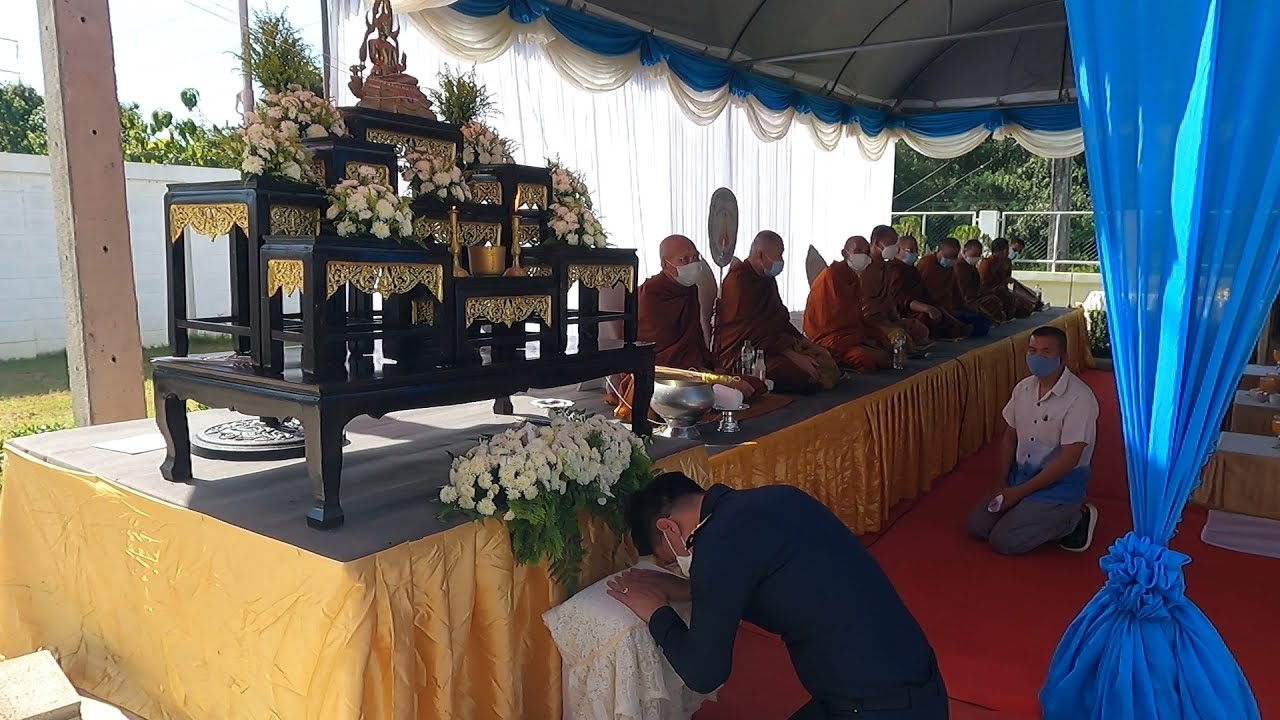The image depicts an outdoor Buddhist ceremony or homage taking place on a sunlit patio with a distinctive red floor. Central to the scene is a black altar adorned with statues and white flowers. A man in a suit is kneeling in a position of reverence in front of the altar. To the right of the altar, several monks in red and orange robes are sitting cross-legged on a black stage draped with gold fabric accents. All the monks are wearing white face masks. Behind the kneeling man is another individual, wearing a white polo shirt and blue pants, also kneeling directly on the red floor. The setting is framed by a blue curtain tied at the bottom and a white curtain hanging behind the monks. Adjacent to the altar is a concrete pillar, and the entire scene exudes a sense of solemn dedication and spiritual reverence amidst ceremonial decor.